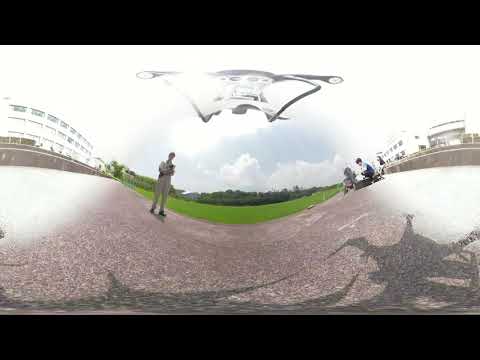On a bright and slightly cloudy day, an image showcases a bustling skate park and adjacent green space. In the foreground, a man stands on gray cement pavement, holding a controller to navigate a camera drone that hovers near the top center of the image. The scene captures the distortion and vibrant colors, typical of a fisheye lens effect. To the right, two kids sit next to a skateboard, intently watching the drone activity. The background reveals grass and trees, hinting at a park-like area. Additionally, on both the left and right sides, large white and gray buildings with ample glass windows frame the scene, further enhancing the urban park setting.